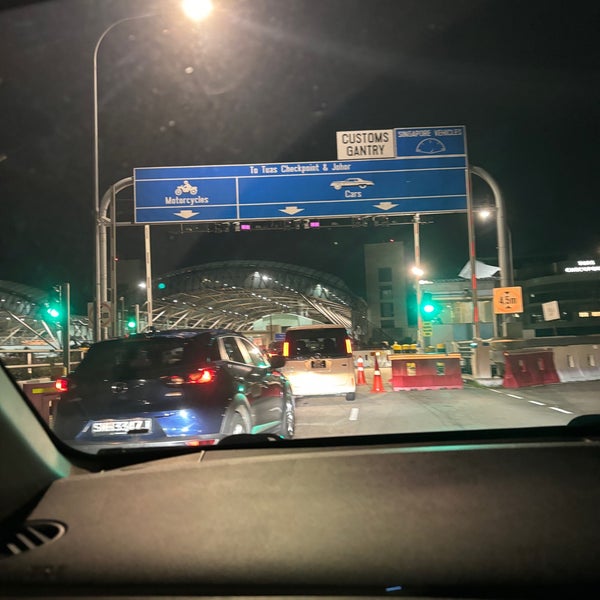The photograph depicts a small traffic jam at night, just before a customs checkpoint on a roadway, likely at a border crossing in a European or Middle Eastern region. The image was taken from inside a vehicle, showing part of the dashboard. Above, there is a prominent blue sign indicating different lanes: the far left for motorcycles and the middle and right lanes for cars. Additionally, there is a white sign labeled "Customs Gantry," and other signs that partially read "Signaport Vehicles" and an incomplete "to TE" phrase. The scene includes an open-air arch structure illuminated by ample street lights, clearly marking the checkpoint. Two vehicles are directly ahead: an SUV with a blue paint and a white utility vehicle. The rightmost lane is blocked off by orange barriers. The stoplights above are both green, signaling that the vehicles at the front are ready to move forward.